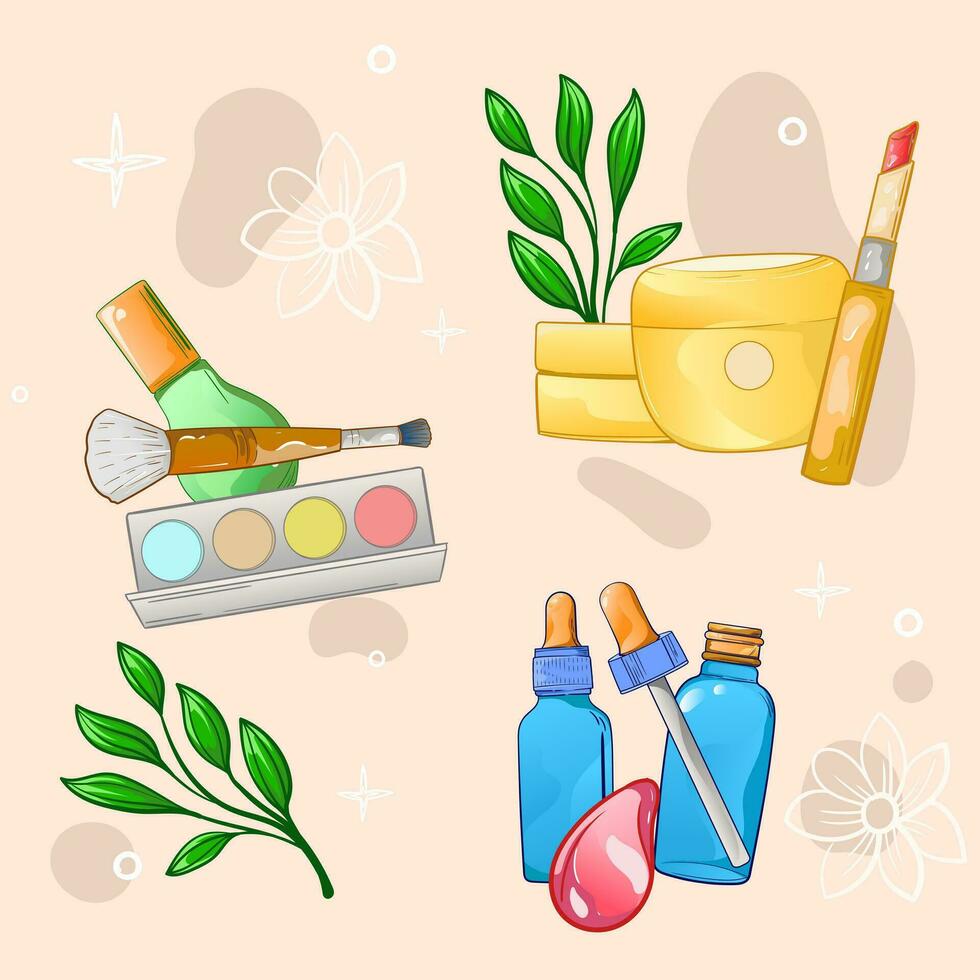This digitally-generated animated image features a captivating collage of various products set against a pinkish-beige canvas background adorned with blurred white flowers, abstract star patterns, and cylindrical shapes in white and brown. Prominently displayed are colorful illustrations of different items: towards the left, a yellow jar accompanied by a matching yellow flower vase holding a green plant, as well as a dual-sided makeup brush with blue, brown, yellow, and pink eye shadow in round compartments. A green bottle with a gold cap is situated below the brush. Adjacent to these, on the upper right, there is a small knife, which appears to double as a colored pencil, a compact paintbrush and a bottle of cream or lotion with leafy decoration. The scene also includes a compact makeup kit with an assortment of colors and a green bulb. Further down, on the bottom right, sit two blue jars with eyedropper-style lids, flanking a small, reflective red droplet. Sprinkled throughout are illustrations of green leaves and stems, enhancing the artistic and whimsical nature of the composition. This vibrant array vividly showcases a variety of artistic and cosmetic tools against a seamless and surreal background.